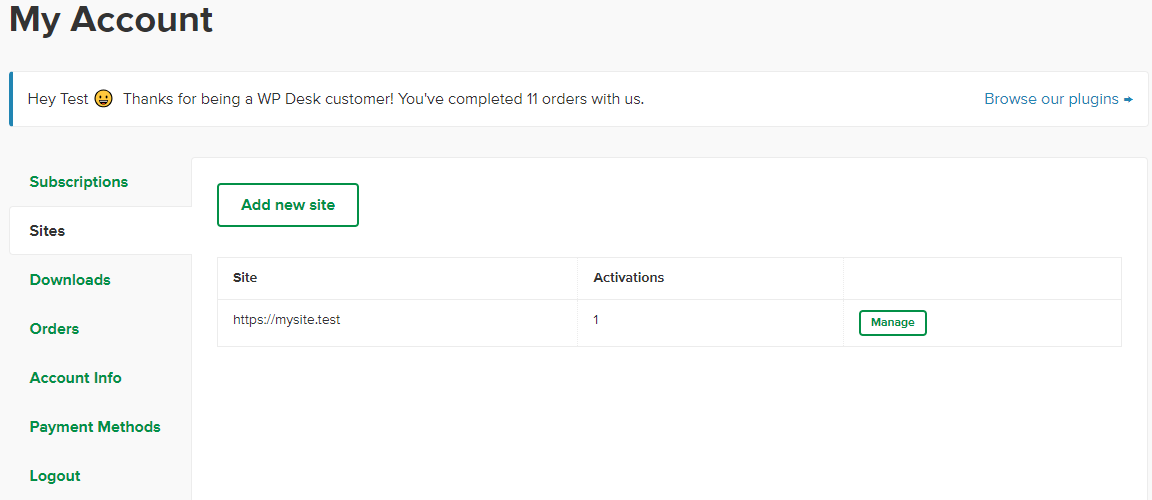This image depicts a "My Account" page with various user interface elements and features. 

At the top, there's a banner displaying a message with the text: "Hey, test 😊 Thanks for being a WP Desk customer! You've completed 11 orders with us." To the far right of the banner is a right-facing arrow, indicating an option to browse plugins.

Below the banner, there is a darker, faint gray section with tabs organized for easy navigation. These tabs include: Subscriptions, Sites (which is currently selected), Downloads, Orders, Account Info, Payment Methods, and Log Out. All tab labels are in green text.

The main content area below the navigation tabs is white. The user is on the "Add New Site" section within the Sites tab. This section displays a section with four labeled boxes. The first box, labeled "Site," contains the URL "http://mysite.test." To its right, within the second box labeled "Activations," is the number "1." 

Below these boxes, a green-outlined button with green text labeled "Manage" is visible, providing an option to manage the site.

Overall, the page offers a clean and organized layout for managing account details and site-specific options.